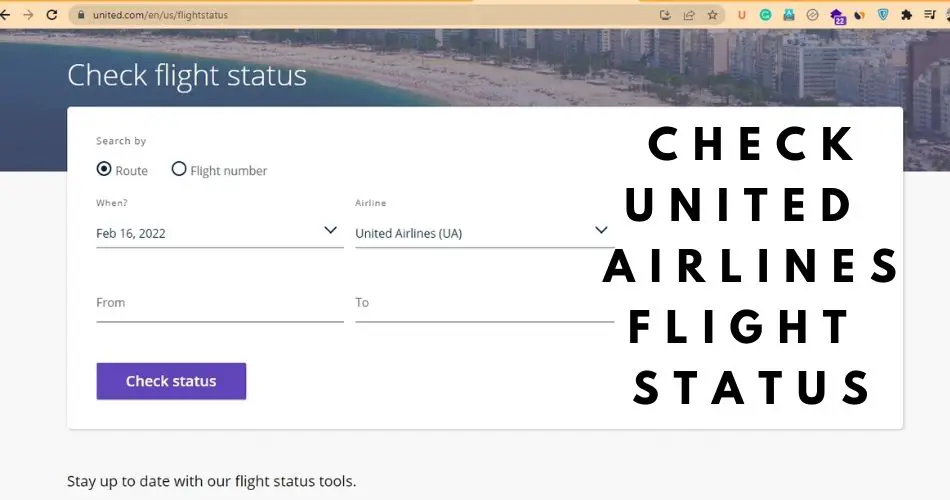The image displays a flight status interface with multiple icons and information. On the top, there are left and right arrows, a refresh icon, and another miscellaneous icon. The main section features status indicators for United Airlines and Canada Airlines flights. The interface includes icons labeled "UG" and the option to check flight status. Visuals include a background image of a beach with skyscrapers, accentuated with elements that appear purplish. There's a search function that allows users to check routes and flight numbers. A black section confirms checking the status of a United Airlines flight departing on February 16, 2022. The layout features a blue bar for checking status, a gray-edged interface, with a red down indicator, a green shield icon, and what appears to be a puzzle piece. The bottom section encourages staying updated with flight status tools.